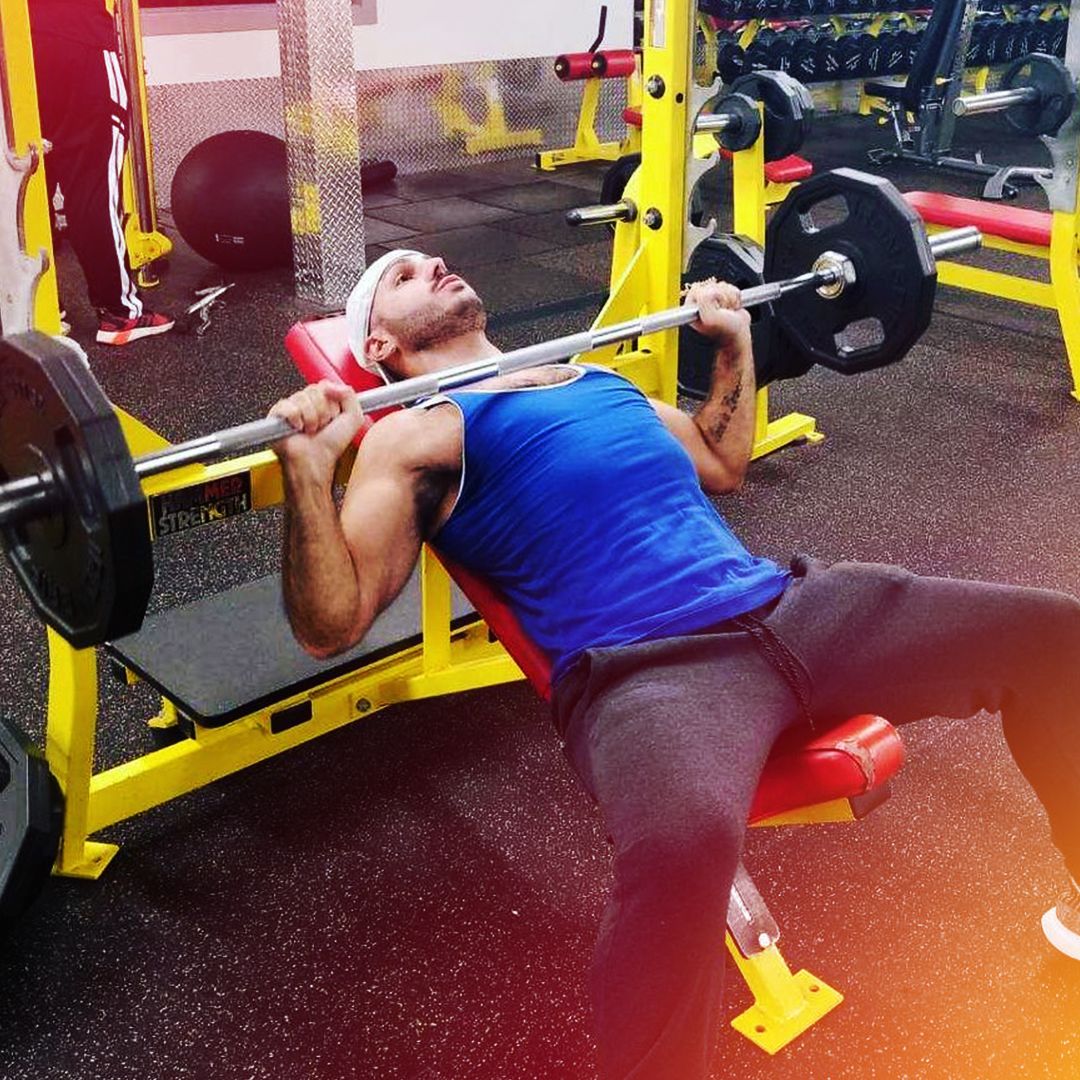The image depicts a fairly young man, around 30 years old, working out alone in a gym. He is using a chest press machine with a yellow frame, and a red bench that features silver and yellow metal accents at the base. The man is in the process of performing a bench press; the bar, which is silver with dark gray weights at each end, rests against his chest just below his neck. He is dressed in a blue tank top with white outlining near the collarbone area, dark gray sweatpants, and tennis shoes, though the shoes are mostly cut off in the image. A white baseball cap is worn backwards on his head. The gym has a black floor speckled with white, and the background includes various gym equipment like free weights on a holder, a big black fitness ball, and red and yellow machines. There is another person partially visible in the upper left-hand corner, identifiable by their red and black sneakers and black pants with white stripes.